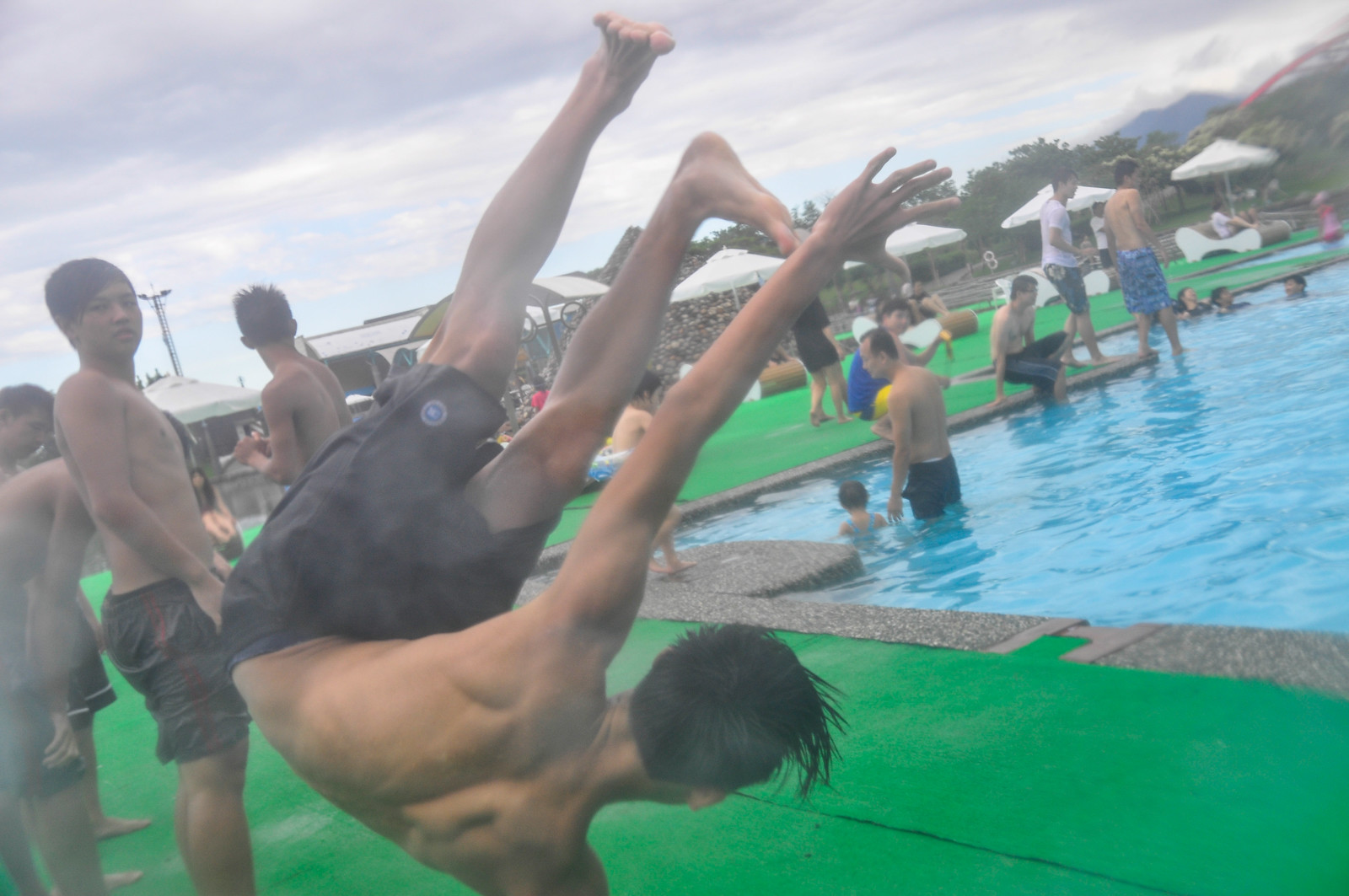The image depicts a bustling outdoor public pool area on a cloudy day. The pool is situated to the right, with numerous people, including young men and children, both in and around the water. The poolside is lined with pristine white umbrellas and lounging chairs, providing a place for relaxation. The ground surface around the pool is green, possibly soft turf or standard pool decking. In the foreground, a boy with short black hair and black swimming trunks is performing an impressive one-handed handstand, with his legs and free arm extended into the air. To his right, another boy with similar black hair observes the scene, adding to the lively atmosphere. In the background, trees and scattered clouds frame the scene, completing this snapshot of a day at the public pool.